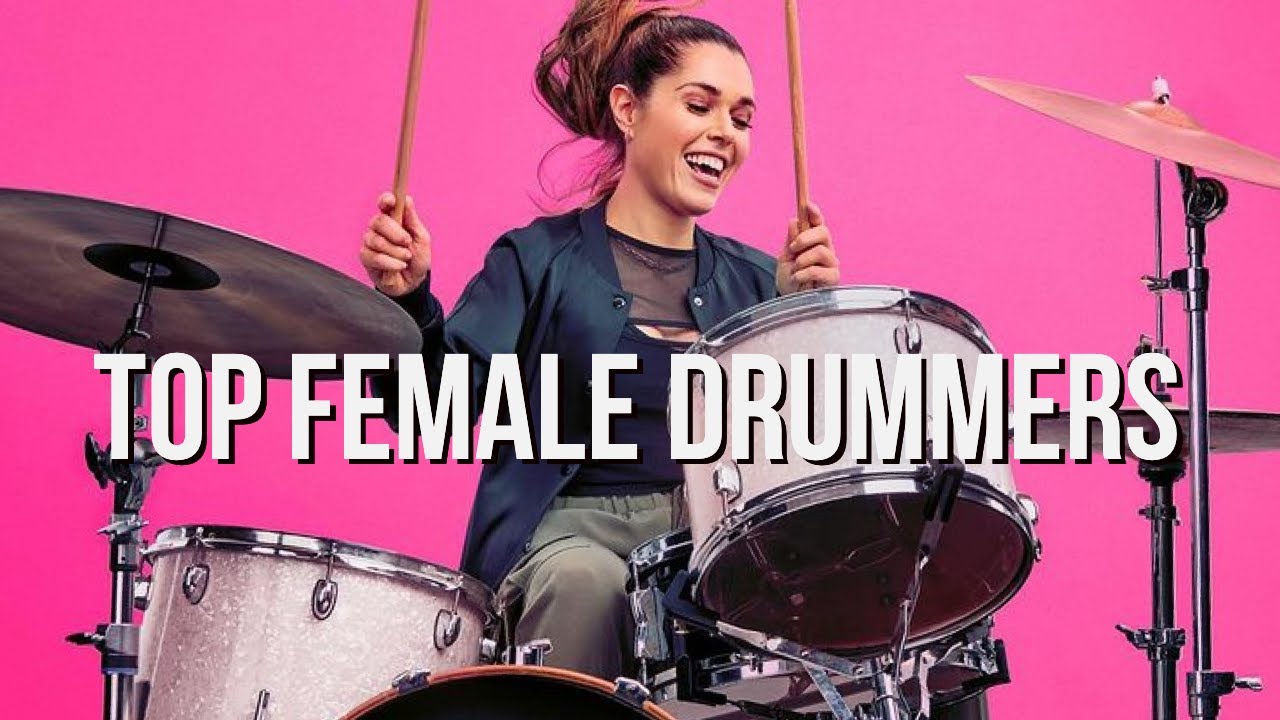In this vibrant thumbnail from a YouTube video, Domino Sant'Antonio is captured mid-performance with a beaming, joyful expression, her eyes closed and mouth open in a wide smile. She is a recognizable figure from the Drumeo YouTube channel. Positioned against a vivid pink background, she sits behind a striking white ivory drum kit with sparkling silver sides, equipped with cymbals on both the left and right. Her brown hair is pulled back into a loose bun, neatly away from her face. Domino is dressed in a dark top, light gray pants, and a dark teal jacket. She holds her pale wooden drumsticks up at shoulder level, ready to strike the drums with enthusiasm. Overlaid across the middle of the image in bold white block text is the title "Top Female Drummers."